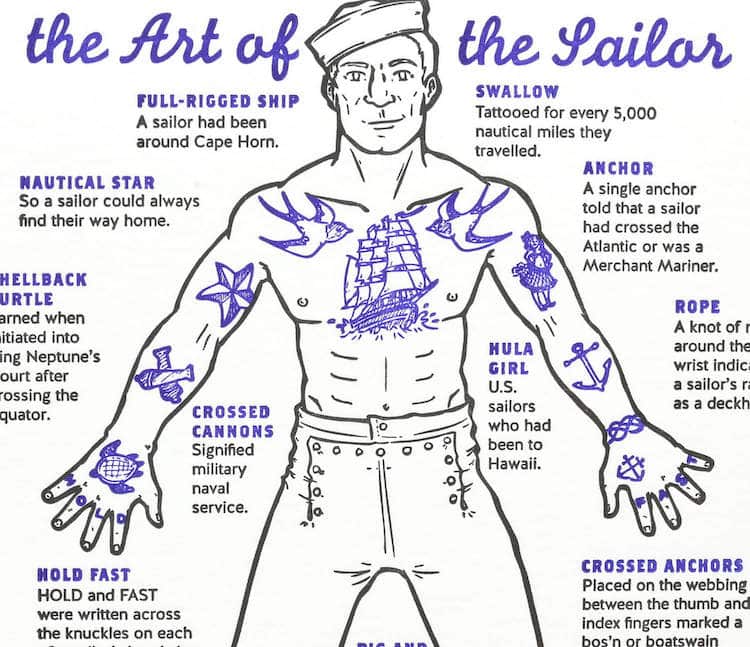This is a detailed hand-drawn, black and white diagram titled "The Art of the Sailor" in a stylish purple script, with "The" and "Of" in lowercase, "Art" with a capital "A," and "Sailor" with a capital "S." The image features a shirtless sailor with arms outstretched, wearing white pants decorated with numerous buttons on a prominent front flap, and a traditional sailor hat. Surrounding the sailor's head, the words "The Art of" appear to the left, and "The Sailor" to the right, both in blue cursive.

The sailor's body is adorned with numerous tattoos, each meticulously labeled to explain its significance. Notably, his knuckles bear the words "Hold" and "Fast" across each hand. Different tattoos indicate various achievements and experiences of the sailor's life:

- **Ship Tattoo**: A full-rigged ship on his chest signifies that the sailor has navigated around Cape Horn.
- **Swallow Tattoos**: Birds on his chest represent every 5,000 nautical miles traveled.
- **Nautical Star**: A star tattoo, indicating that the sailor can always find their way home.
- **Anchor Tattoo**: A single anchor tattoo signifies that the sailor has crossed the Atlantic or served as a merchant marine.
- **Crossed Anchors**: Located in the webbing between his thumb and index finger, these tattoos mark the sailor as a boatswain or bosun.
- **Crossed Cannons**: Found on his lower arm, these tattoos denote experience in naval military service.
- **Turtle Tattoo**: This indicates the sailor was inducted into Neptune's court after crossing the equator.
- **Rope or Knot Tattoo**: Around the wrist, suggesting the sailor's role as a deckhand.
- **Woman Tattoo**: Depicts that the sailor has visited Hawaii.

Additional adornments include a Celtic knot-like cross and other various designs that further enrich the sailor's story and maritime adventures. The detailed labels of these tattoos provide a comprehensive understanding of the sailor's extensive and varied experiences at sea.